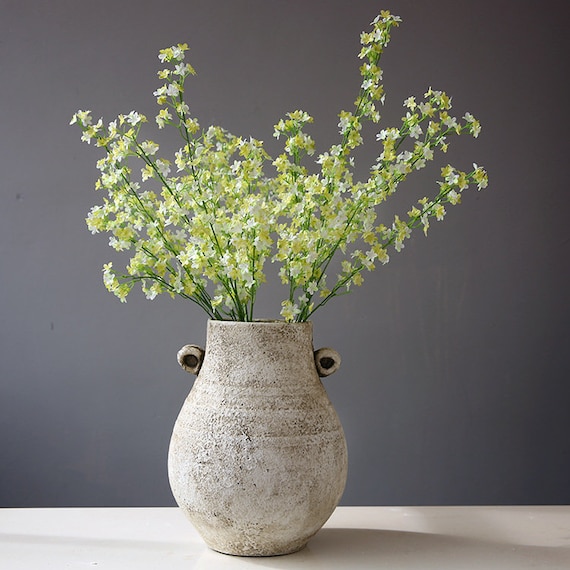The image features a professionally photographed vase with a rustic, antique look, characterized by an off-white, ceramic surface adorned with subtle pockmarks and darkened markings. The vase, somewhat bulbous at the bottom with handles on either side resembling small ears or circles with black centers, tapers towards the top. It rests on a white surface, set against a medium to dark gray background that varies in illumination.

Emerging from the vase are numerous green stems—approximately 15 to 20 in number—each adorned with delicate winter jasmine flowers. These small blossoms predominantly feature pale yellow petals with white accents, some appearing almost entirely yellow due to their minute size. The subtle blending of the green stems with the flowers' soft hues creates a harmonious visual flow as the stems lean gently in different directions.

The overall composition, complete with intricate play of light and shadows, suggests a high level of craftsmanship, possibly intended to market either the vase or the artificial yet highly realistic winter jasmine bouquet within it.